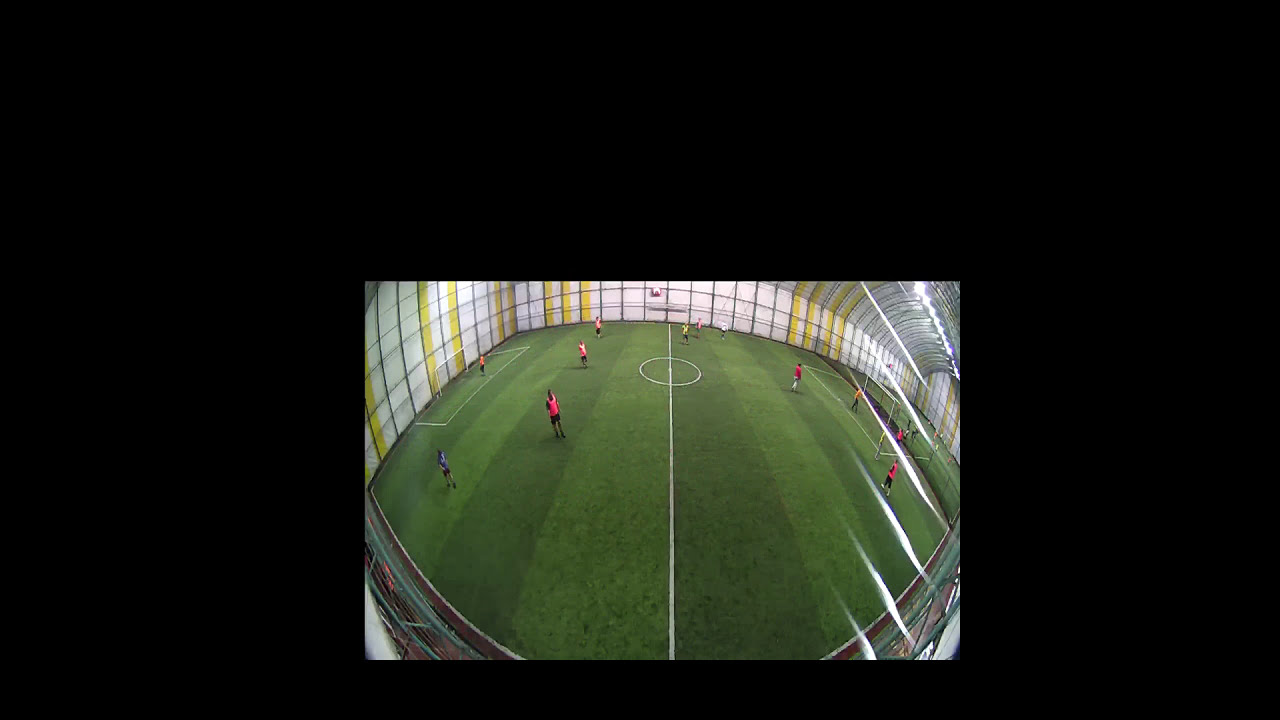The photograph is a panoramic, fisheye lens shot of an indoor soccer field with an artificial grass surface. The field, nestled within a glass-enclosed gymnasium with interspersed white and yellow stripes stretching from the ground to the ceiling, is split down the middle by a prominent white line. On the left side of the image, a team of players donning red jerseys and black shorts is seen, while another team with red jerseys and what seem to be white socks is positioned on the right. This composition suggests the photograph might be the result of two images melded together to create a mirrored, panoramic view. Though the nets are barely visible, their presence is implied on either side of this compact, non-traditional pitch. The image, framed within a larger black background as if highlighted, showcases a color palette of green, yellow, white, black, red, gray, and silver, echoing a realistic style representative of indoor sports photography.